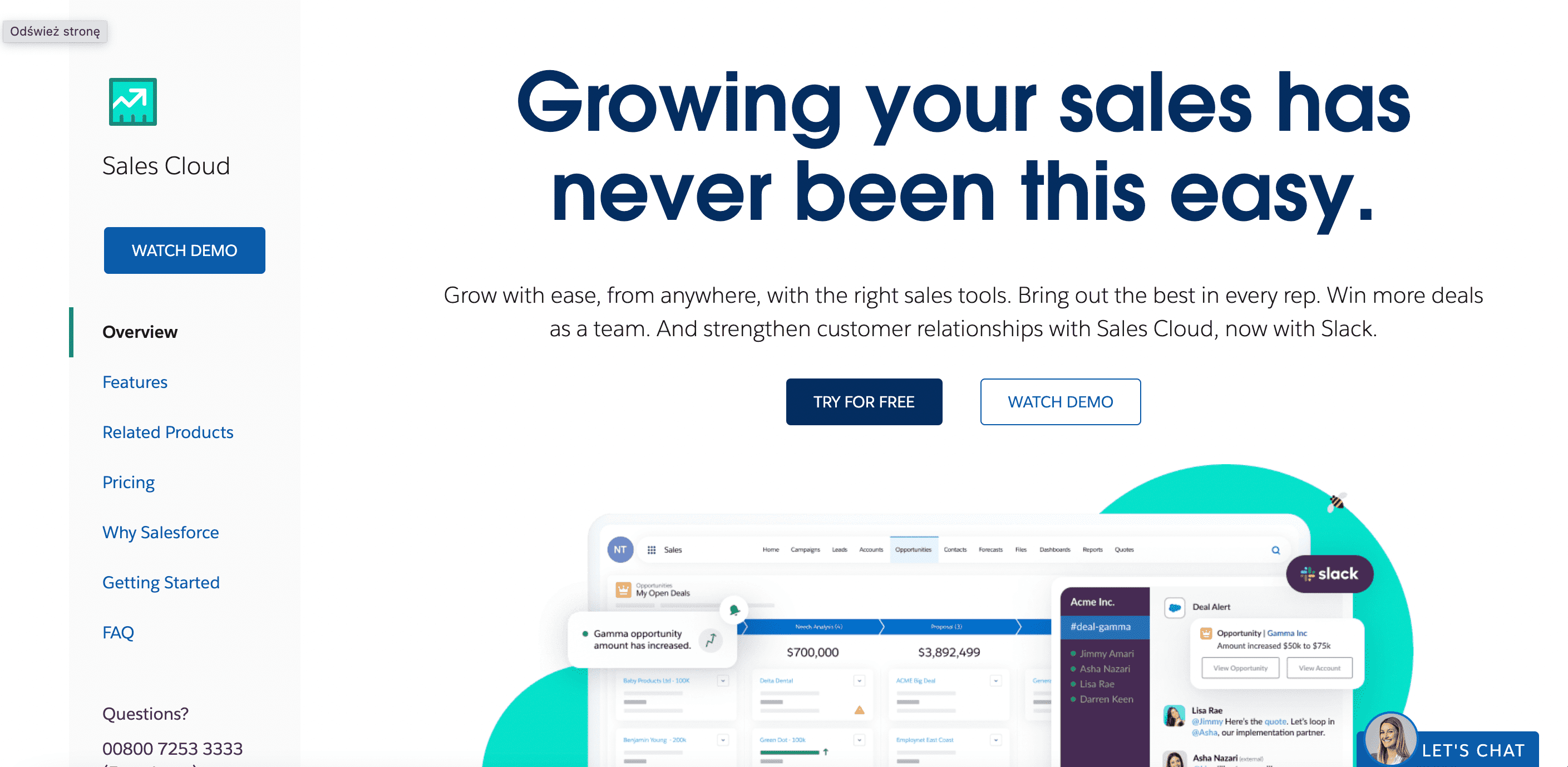The image depicts a screenshot from a website showcasing the features of a sales tool. On the left side, there is a vertical gray banner. At the top of this banner, the word "ODŚWIEŻSTRONĘ" is displayed in various languages. Below this, there is a section enclosed by a dark green outline, featuring a sea-green background and a sales graph with an arrow that moves up, down, and then ascends. Beneath this graph, a blue button with white text reads "Watch Demo." 

The gray banner continues with black text labeled "Overview," followed by a series of blue text links: "Features," "Related Products," "Pricing," "Why Salesforce," "Getting Started," "FAQ," and a "Questions?" section that provides a phone number.

In the main, central white background area, there is prominent black text stating, "Growing your sales has never been this easy." Below this, smaller text elaborates: "Grow with ease from anywhere with the right sales tools. Bring out the best in every row. Win more deals as a team and strengthen customer relationships with Sales Cloud. Now with Slack." 

Two buttons follow this text: one with a navy background that says "Try it for Free," and another that says "Watch Demo." Lower on the page, an image of a computer screen is displayed with various options available for selection.